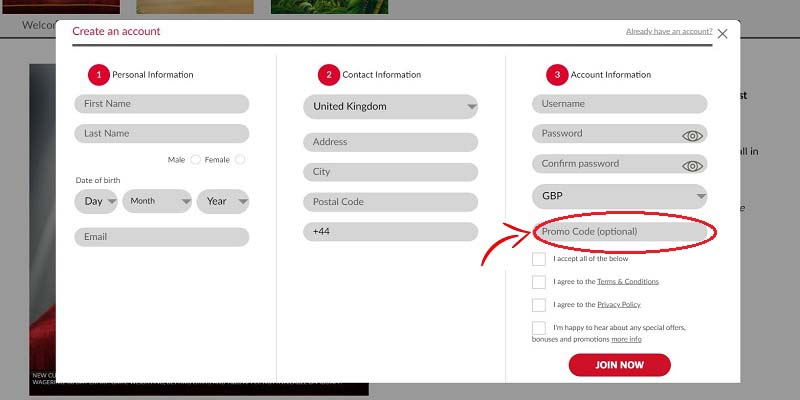The image showcases a webpage with a white background titled "Create an Account" in prominent red text at the top. The signup form is segmented into three main sections. 

1. **Personal Information:**
   - **Fields:** First Name, Last Name
   - **Gender Options:** Male, Female
   - **Date of Birth:** Day, Month, Year
   - **Email Address:** A designated field for entering the user's email

2. **Contact Information:**
   - **Country Selector:** Defaulted to "United Kingdom" with a grey downward-facing arrow indicating a dropdown menu for other regions
   - **Fields:** Address, City, Postal Code
   - **Phone Number Prefix:** Defaults to "+44," the country code for the United Kingdom

3. **Account Information:**
   - **Fields:** Username, Password, Confirm Password
   - **Currency:** Default set to GBP, indicated as a dropdown menu for other options
   - **Promo Code:** An optional field highlighted by a red circle and an arrow pointing towards it

Below these sections, there are several checkboxes with corresponding labels:
- "I accept all of the below"
- "I agree to the Terms and Conditions"
- "I agree to the Privacy Policy"
- "I'm happy to hear about any special offers, bonuses, or promotions"

A "More Info" button is available for additional details. The form concludes with a prominent "Join Now" button in white text set on a red background. Most of the text and input boxes on the page are styled in white and grey.